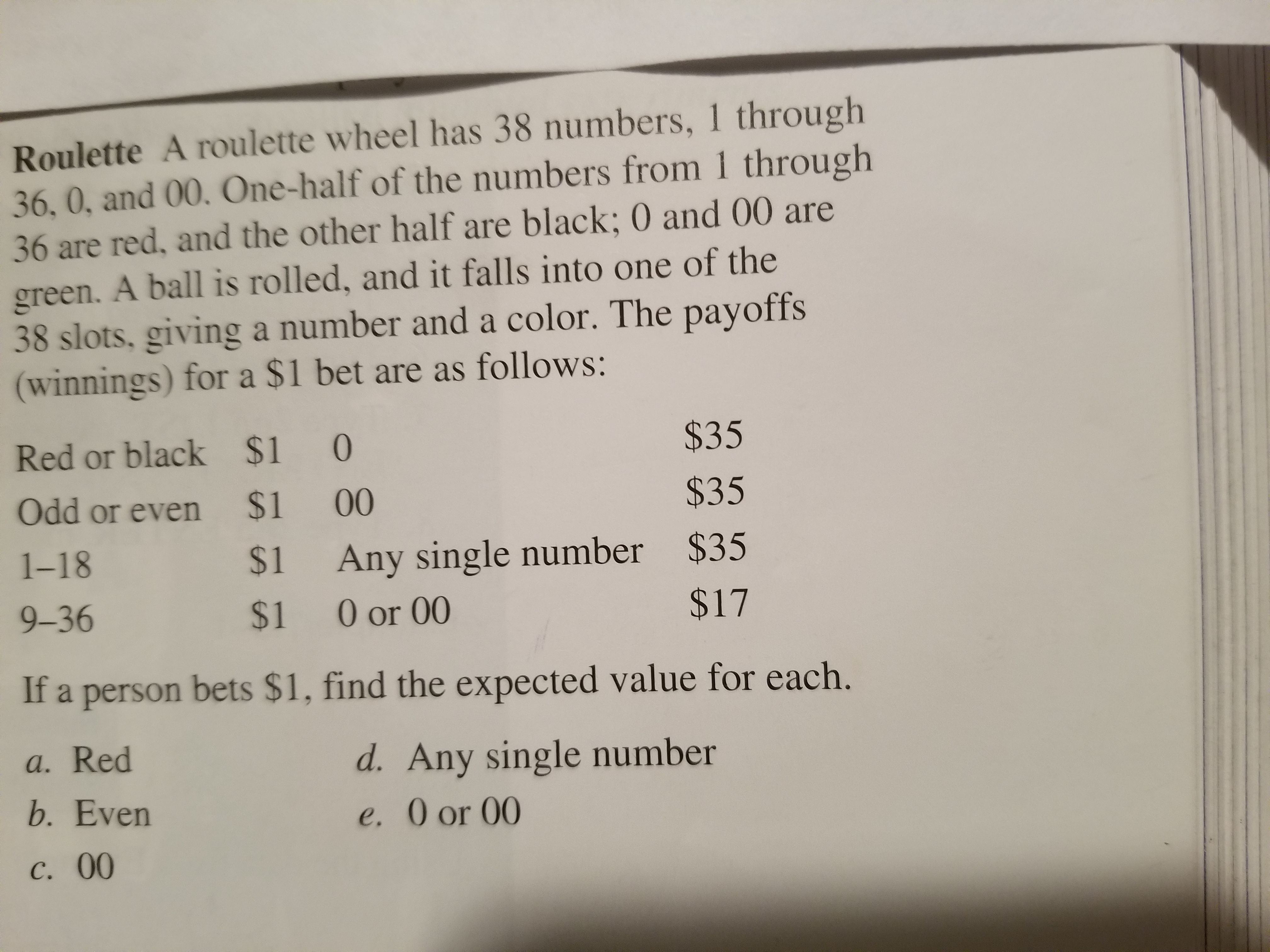The image depicts a detailed black-and-white close-up of a page from a thick textbook. The visible text on the page, positioned on the right side, is topped by the bold heading "ROULETTE". Above this page, the back of the book and the thickness of its pages are clearly visible. The page itself delves into the mechanics of roulette, explaining that the wheel features 38 numbers: 1 through 36, 0, and 00. Numbers 1 through 36 are split evenly, with half red and half black, while 0 and 00 are green. It describes that a ball is rolled, landing in one of the 38 slots to determine a number and a color. The payoffs for a $1 bet are listed as follows: red or black, $1; odd or even, $1; numbers 1 through 18, $1; numbers 9 through 36, $1; 0, $35; 00, $35; any single number, $35; and a combined bet on 0 or 00, $17. The page concludes with a question prompting the reader to calculate the expected value for a $1 bet on various outcomes: A. Red, B. Even, C. 00, D. Any single number, and E. 0 or 00. Some shadows are cast halfway down the page, adding to the depth of the image.